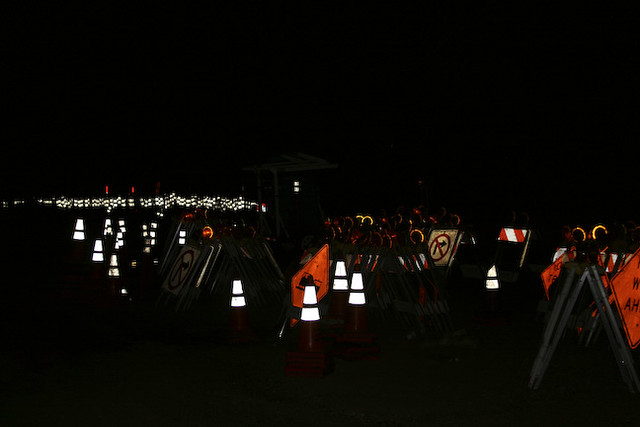Against a stark black background, a collection of road signs and construction cones stand prominently. The white and orange colors of the signs and cones contrast sharply with the dark backdrop, creating a striking visual effect. The array of signage, which includes various work and warning signs, suggests a scene set amidst a construction zone or roadway maintenance area. The overall setting evokes a sense of caution and alertness, as if captured in a moment of paused activity on a bustling worksite.